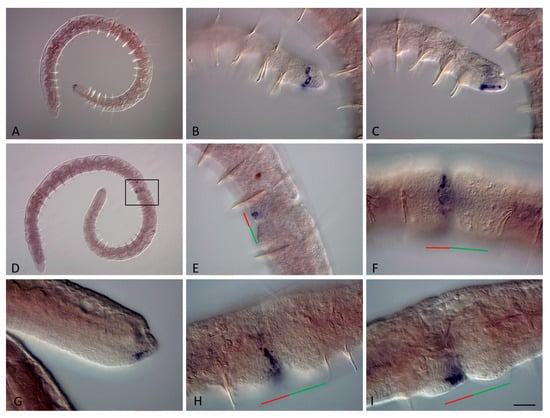This image is a detailed collage of nine photos, arranged in three rows and three columns, each labeled with letters A through I in the bottom left-hand corner. The collage features a sequence of progressively zoomed-in views of what appears to be a pink, swirled organism resembling a worm, possibly viewed under a microscope. 

The photos all share a gray background and depict different magnifications of the worm-like organism. Photo A and D present more distant views of the entire worm, while the intermediate photos (B, C, E, F, G, H, and I) offer closer examinations. Key details, such as two black spots near the head and a distinguishing red and green line appearing in several zoomed-in views (specifically E, F, H, and I), are highlighted throughout the collage. As you move from left to right and top to bottom, each photo provides increasingly detailed closeups of these features, culminating in the bottom row, which displays the most magnified images, focusing on the worm's head and the contrasting line. This collage effectively illustrates both a macroscopic and microscopic perspective of the worm-like organism.